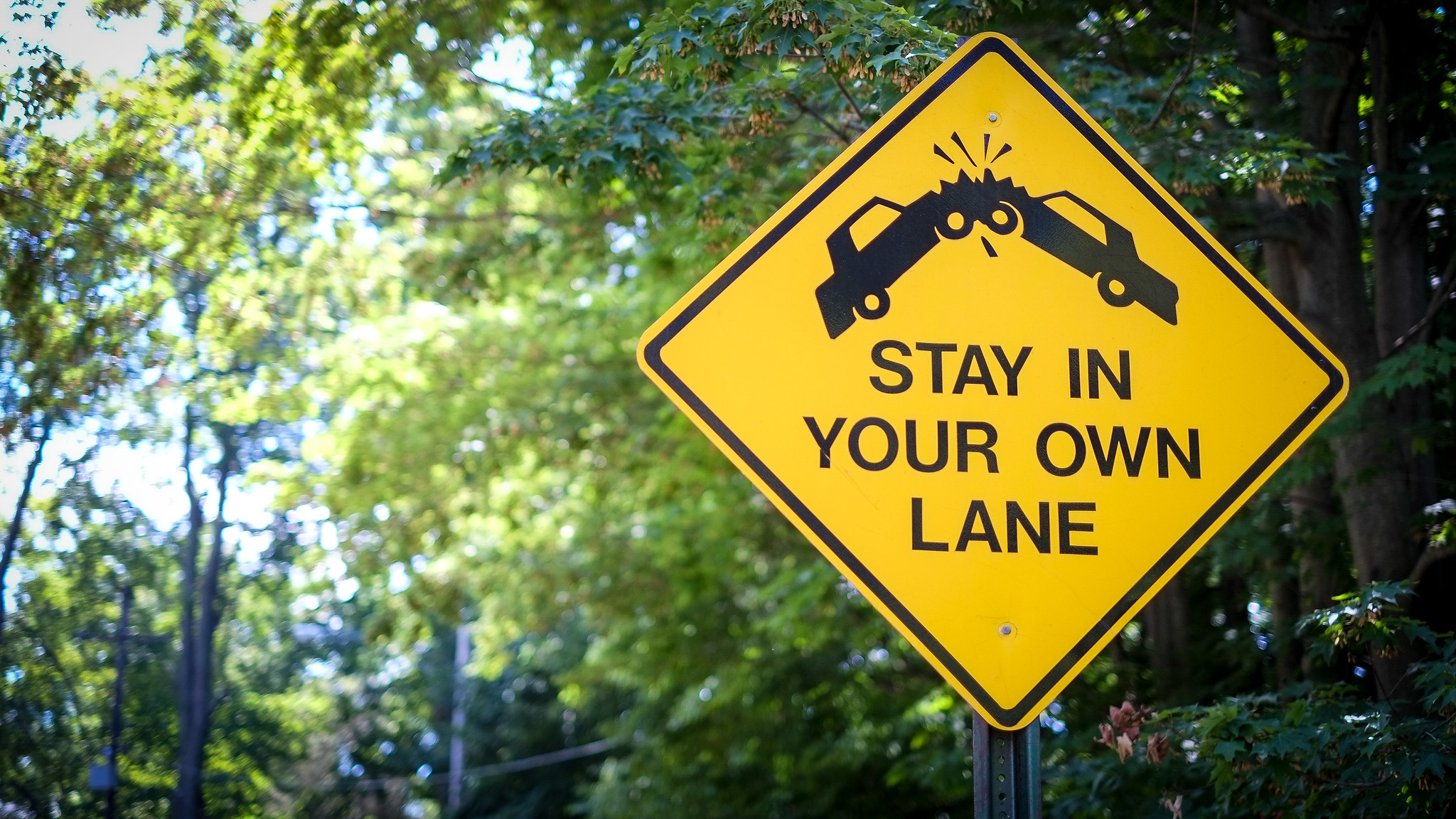In this photo, a diamond-shaped, yellow traffic sign is prominently displayed against a backdrop of vibrant trees in what appears to be a warm, sunny spring or summer day. Rays of sunlight filter through the green and yellow foliage, further illuminating the sign. Mounted on a metallic green pole, the sign features a thick black border and a central illustration of two black cars colliding, their front ends lifted slightly off the ground. Black lines radiate from the point of collision, accentuating the impact. Below the image, in bold, capital letters, the sign instructs, "STAY IN YOUR OWN LANE." The sign, elevated and clear, serves as a stark warning amid the serene natural setting.